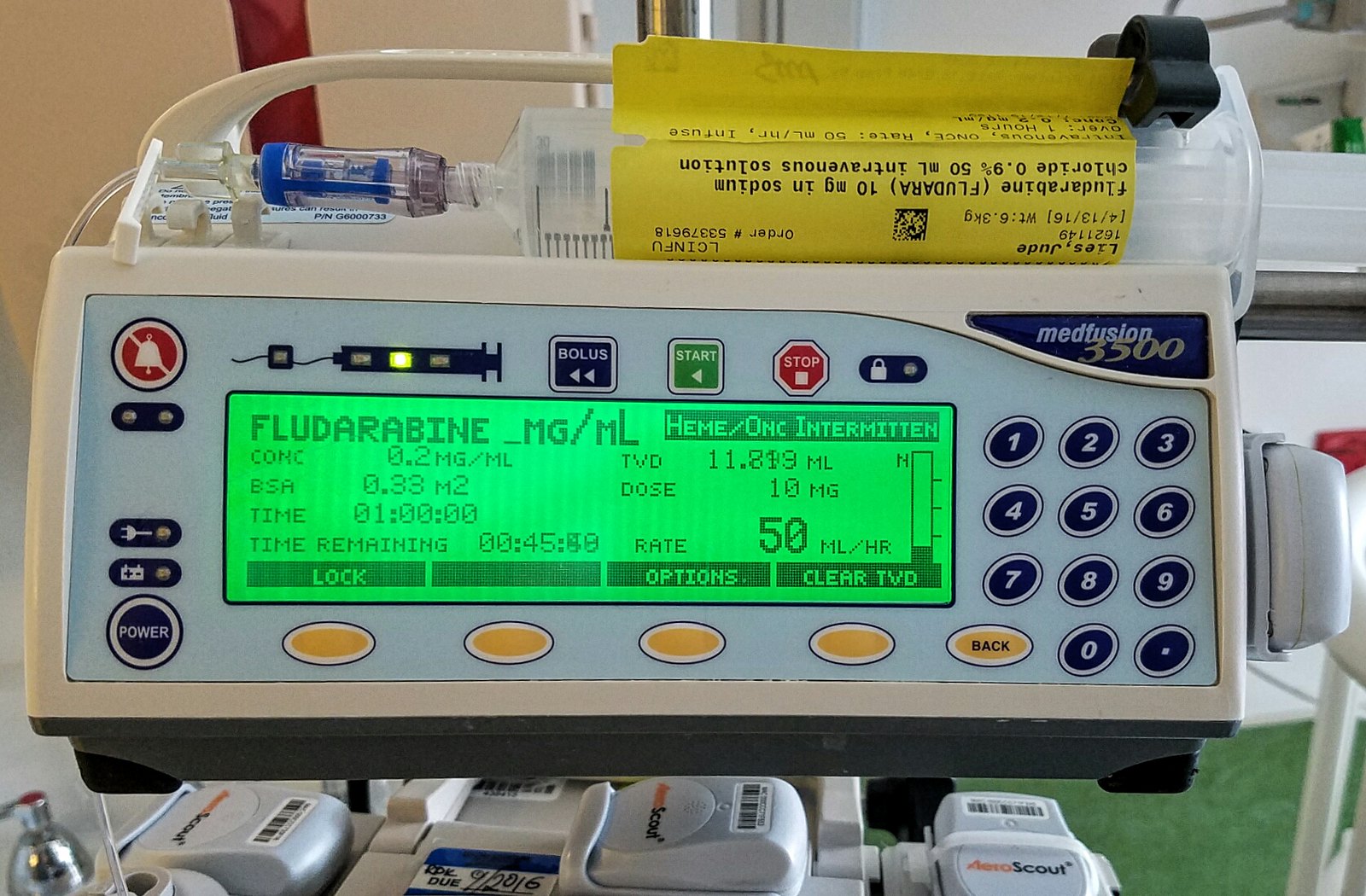This detailed, close-up color photograph showcases the MedFusion 3500, a medical infusion device commonly used in hospitals to regulate intravenous medications. The device, white and approximately the size of a small home printer, features a prominent green LED display in the center with black text. The screen reads: "FLUDARABINE MG/ML HEMI-ONC Intermittent," along with dosage information such as "0.2 mg/ml BSA 0.33 m2," and the current infusion rate of "50 milliliters per hour." The timer indicates "time remaining 45 minutes and 40 seconds."

Attached to the top of the device is a large plastic syringe filled with fluid, labeled with a yellow piece of paper. The label, though upside down, details the medication as "Fludarabine 10 mg in Sodium Chloride 0.9%, 50 milliliters intravenous solution." The syringe connects to a tube that extends out the left side of the machine.

The control panel to the right of the display features a keypad designed like a telephone, with buttons labeled 0 through 9. Additional buttons include a red circle with a bell crossed out, a green "start" button, a black "bolus" button with two white arrows, and a yellow "back" button. Below the screen, there are five oblong yellow keys, four of which are blank, and labeled buttons like "back" are found under the number pad and used for various functions. A power button is located on the left-hand side of the device. The image focuses on the front section of the MedFusion 3500, highlighting its interface, labels, and attached syringe.